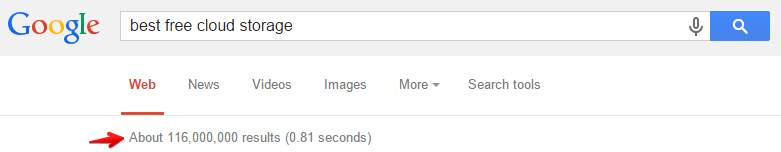A detailed description could read like this:

The image depicts a Google search results page. At the top left corner is the iconic "Google" logo, featuring the uppercase "G" in blue, followed by the letters "o" (red), "o" (yellow), "g" (blue), "l" (green), and "e" (red). To the right of the logo is Google's microphone icon for voice search, a blue square icon that seems to represent a grid or menu, and a magnifying glass symbolizing the search function. Below the search bar are the search category options: "Web" (which is underlined indicating it is currently selected), "News," "Videos," "Images," and "More." There is a right arrow for additional options.

Right beneath these categories is the search results information, displaying "About 116 million results (0.1 seconds)." The background of the page is predominantly white, enhancing the readability of the text and the prominence of the Google logo and icons.